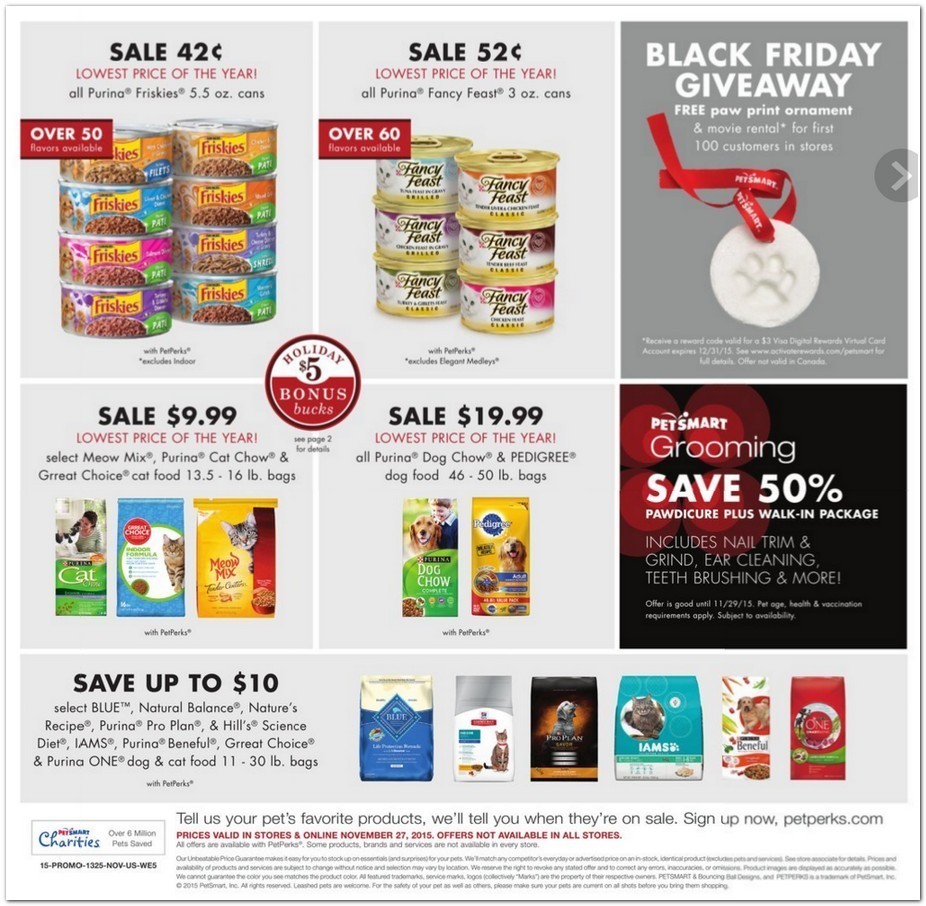**Detailed Caption:**

The screenshot is from the PetSmart website and prominently features multiple savings offers and coupons. The layout is organized into rows and boxes, each box highlighting a specific deal.

In the first row, there are three boxes. The first box features a sale offering Purina Friskies at 5.5 ounces per can for just 42 cents, marking the lowest price of the year. Key details include "42 cents" in bold black lettering and "Lowest price of the year" in attention-grabbing red text. It also mentions "All Purina Friskies" and emphasizes the offer for "over 50" cans in red.

In the second row, the first box showcases another sale, this time for Purina Fancy Feast at 3 ounces per can for 52 cents, similarly noted as the lowest price of the year in striking red letters. Additionally, it highlights a special Black Friday giveaway in a separate box. The giveaway features a free paw print arrangement, illustrated with a circular medallion-like design - a white circle with a paw print, all tied with a red string.

Further down, more coupons are visible. Directly below the Black Friday giveaway, there's an offer for PetSmart grooming services, advertising a 50% discount on a "Paw Declaw Paws Walk-in Package," which includes nail trim and grind services. Finally, the screenshot mentions savings of up to $10 on various pet foods, ensuring a comprehensive range of discounts for different pet care needs.